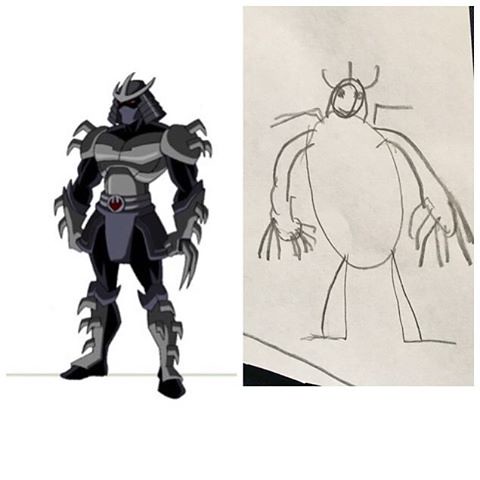Side by side, these two images depict a fascinating contrast between a child's imaginative attempt and the original character from which the inspiration was drawn. The illustration on the left showcases a vibrant, yet roughly sketched children's drawing, aiming to replicate the fierce warrior on the right. The character in the original image is clad in imposing metal armor, adorned with an array of intimidating blades and knife-like features. Though presumed to be a villain, identified by the menacing visage and ornate, cold metal mask, the child artist makes a laudable effort. The youthful drawing captures key details like the stature, the sharp, bladed elements, and the overall aura of the imposing figure, showing a commendable attention to the essentials despite the playful, imprecise style.